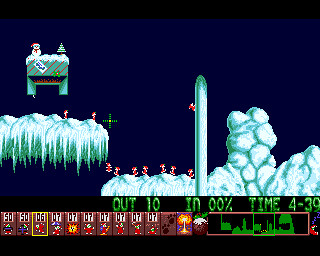The image appears to be a screenshot from a 2D side-scrolling platformer video game. The scene is set against a main dark blue background that gives a sense of depth and atmosphere. The ground terrain consists of multiple levels, primarily depicted in white areas that resemble ice or snowy boulders. Scattered across these icy platforms are approximately 9 or 10 small red characters, which bear an elf-like appearance.

In the top left quadrant of the screenshot, an isolated white platform features a gray base with red stripes. Atop this platform stands a small snowman adorned with a red Santa hat, adding a festive touch to the scene. Directly below this, there is a shorter white platform extending horizontally, adding to the layered complexity of the level design.

Towards the bottom right of the image, a longer white platform is visible, distinguished by having a tall white pole extending upwards from it. This setup contributes to the game's vertical and horizontal navigational elements. The entire scene is anchored by a dark brown border running across the bottom, which likely serves as the ground level or a boundary within the game.